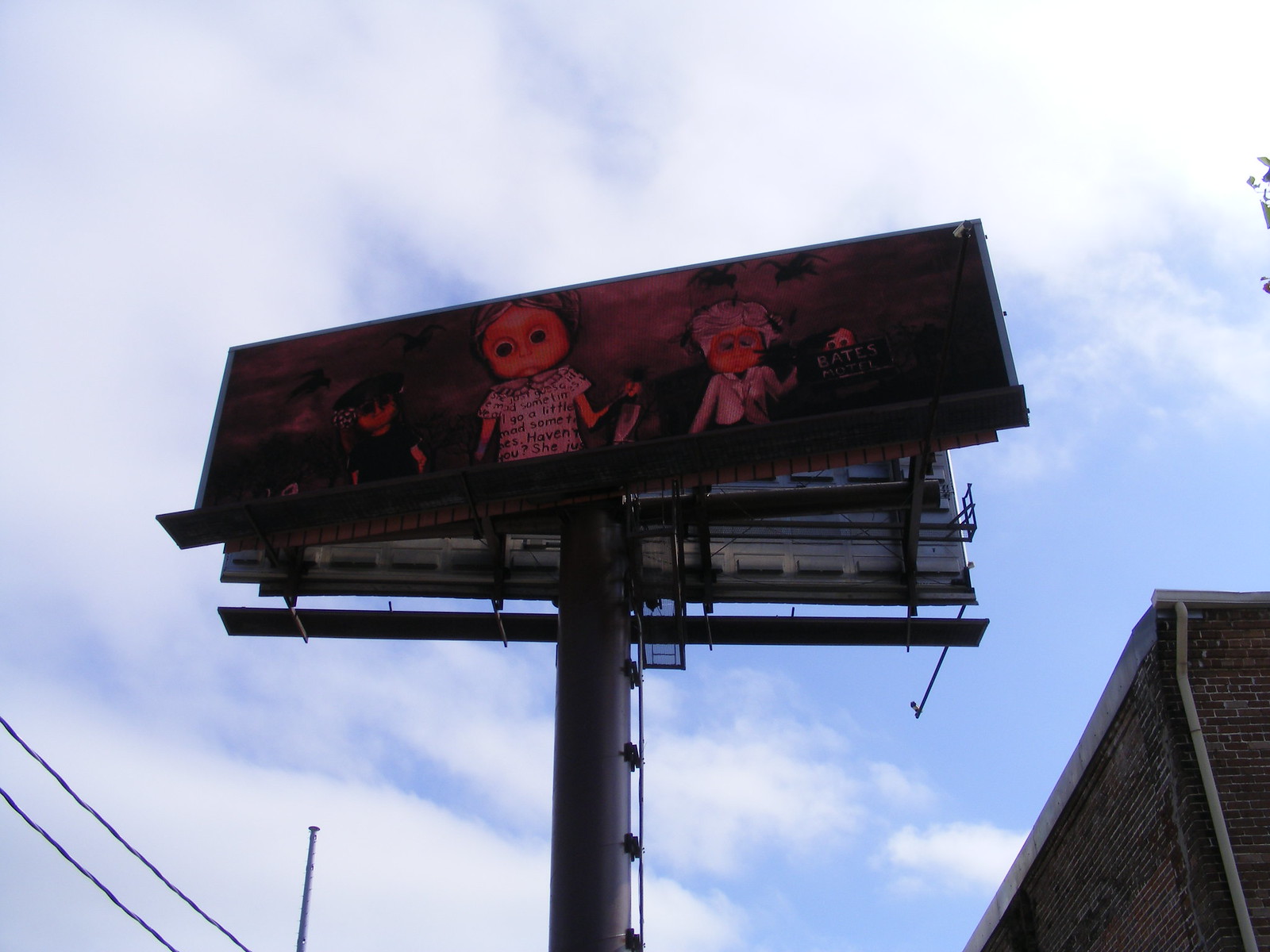In this outdoor daytime photograph, we're looking up at a partially cloudy sky, with a 45-degree camera angle capturing a prominent billboard. The billboard, slightly underexposed due to the backlit conditions, dominates the center of the image and is supported by a massive, smooth pole, resembling a chiseled tree trunk. Positioned above the roofline of a brick building seen on the right, the billboard extends into a sky where patches of blue peek through predominately white clouds. In the lower left corner, crossing diagonally to the right, are utility lines, while a flagpole stands unadorned nearby.

The billboard itself presents two cartoon characters rendered in a horror or fantasy style. On the left side, nearly centered, is a child-like figure with a round face, oversized eyes, a sad expression, and a bald head. This character wears an off-white shirt with the partially discernible words "MAD" and "HAVEN'T." To the right, an older figure with gray hair and red glasses, possibly resembling a grandmother, is dressed in a white dress shirt and appears to be holding a sign that faintly reads "Bates Motel." A second, smaller billboard is visible in the background. The overall scene suggests the advertisement is promoting a dark, possibly animated, series or film.